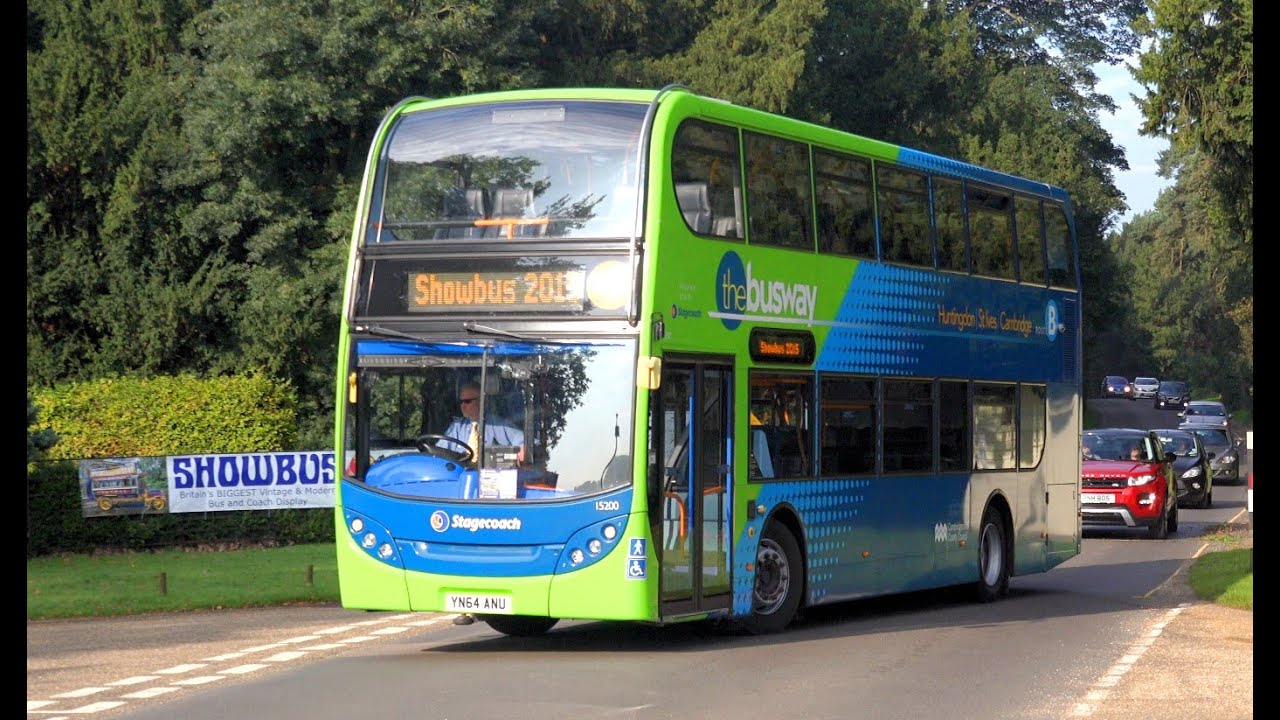This is a photorealistic, horizontally aligned image of a modern double-decker bus turning right on a narrow, single-lane, paved road in a European setting, suggested by the license plate style. The bus is prominently centered in the photograph and exhibits a vibrant color scheme transitioning from green at the front to light and dark blue towards the rear. The front section includes the Stagecoach logo and a blue grille. A light-up sign on the front displays "SHOW BUS 201," with the remaining digits partially obscured by windshield glare. Just below the windshield, and on the side, the bus bears “busway” in white text. The bus appears empty except for a driver dressed in a blue shirt and yellow tie, seated on the right side. Behind the bus is a line of small cars, including a red car followed by several black and gray ones, seemingly stuck in traffic caused by the bus. The road is bordered by dense tree cover and greenery, with only a sliver of sky visible above. Additional details include a white and green banner on the side of the road that reads "SHOW BUS."